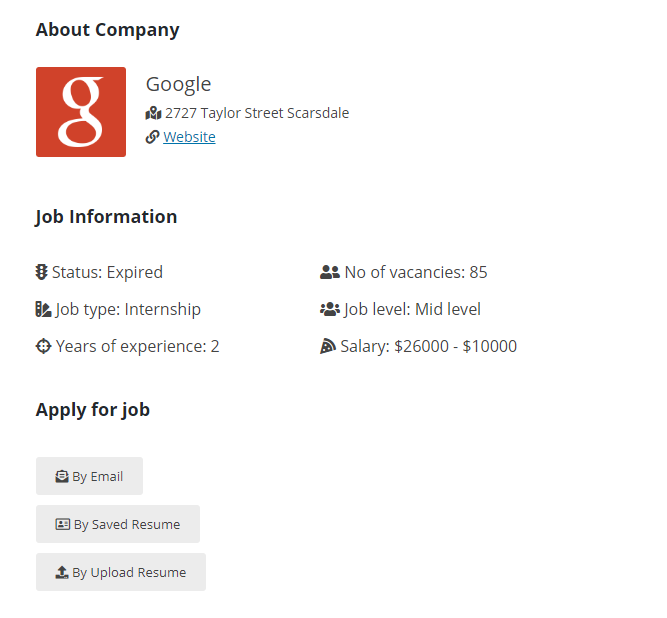The image provides detailed information about a company, specifically Google. At the top, a black header reads "About Company." Directly below, there's a red square with a white 'G' inside, accompanied by the name "Google" in black text. The address "2727 Taylor Street, Scarsdale" is listed beneath.

Further down, there is a link icon followed by the word "website" in blue, underlined text. Next, the section titled "Job Information" includes various job details in black writing: 

- **Status:** Expired
- **Job Type:** Internship
- **Years of Experience:** Two years
- **Number of Vacancies:** 85
- **Job Level:** Mid-level
- **Salary:** $26,000 to $100,000

Notably, there is an image of a pizza next to the word "salary."

The section "Apply for a Job" is outlined below, with three gray rectangular options for application methods:
1. By email
2. By saved resume
3. By upload resume

At the bottom, there are several icons, including a couple representing people, one resembling a stoplight, and another resembling a bullseye.